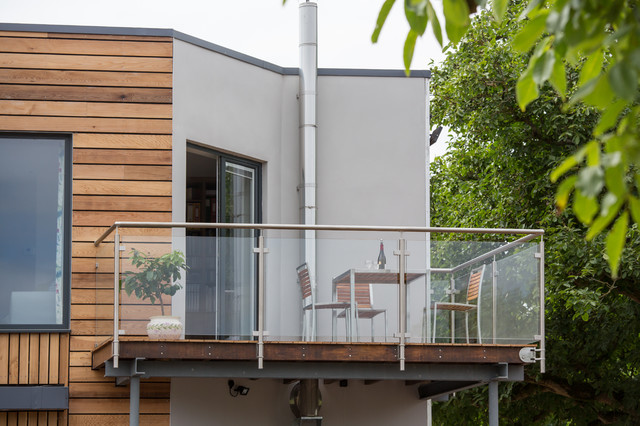This outdoor photograph captures the stylish upper deck of a modern house, featuring a combination of white walls and light beige wood panels. Central to the image is a sleek glass-railed balcony with metal frames, exuding a contemporary elegance. On the deck stands a metal and wood table, accompanied by three matching chairs, clearly styled for outdoor dining. A wine bottle sits atop the table, suggesting a recent or upcoming gathering. To the left of the sliding glass door (which is slightly ajar), a large potted plant in a white pot adds a touch of greenery. Additional verdant elements frame the scene, with trees and bushes on the right and green foliage hanging into the top right corner. The juxtaposition of natural and man-made elements enhances the tranquil yet sophisticated ambiance of this outdoor space.